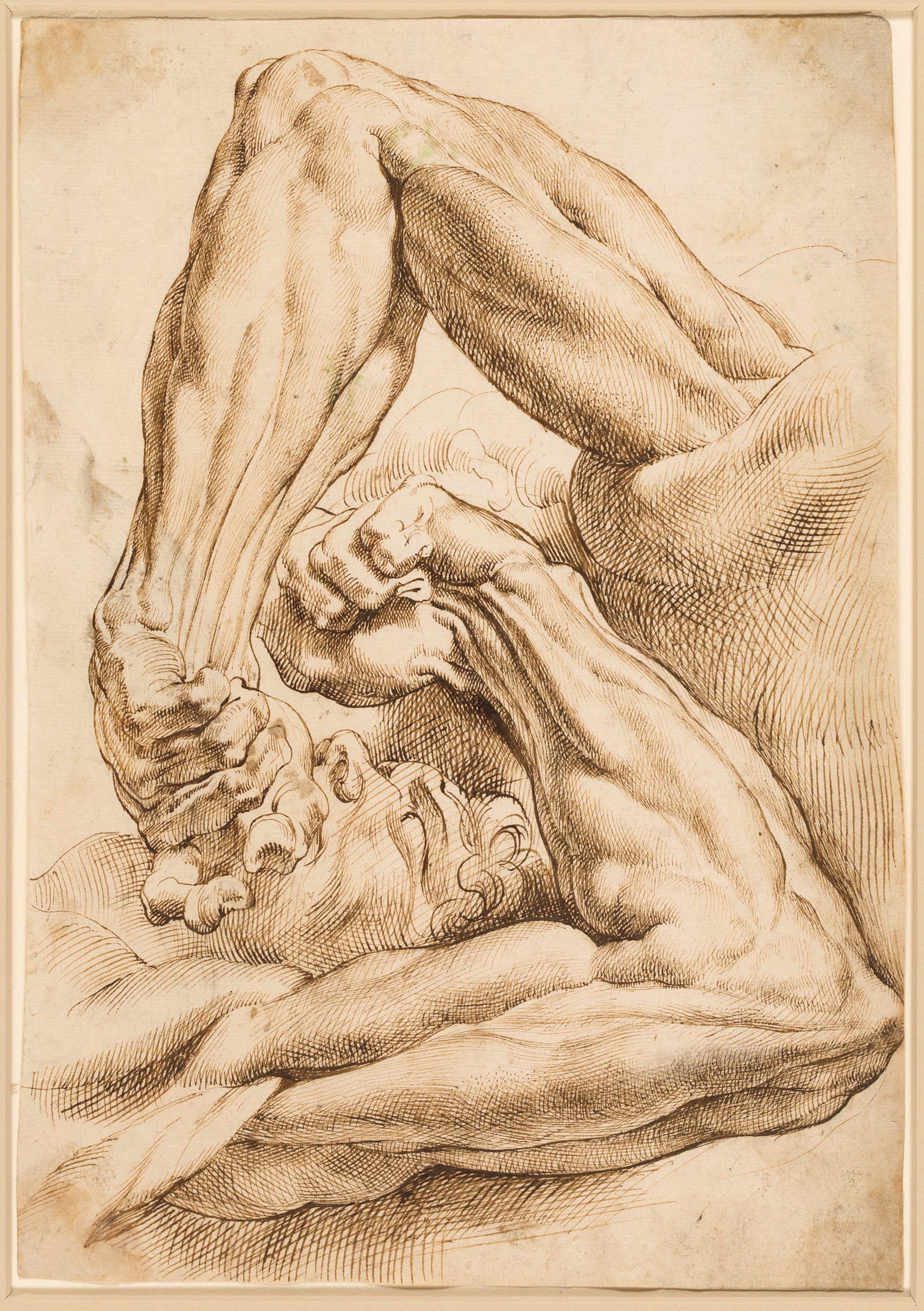In this detailed illustration, the artwork features two intricately sketched arms in dynamic poses. One arm, originating from the left-hand side, extends horizontally before bending vertically upwards at the forearm, culminating in a tightly closed fist positioned at the center of the composition. The second arm, visible with its sleeve, extends upwards before the forearm bends downwards, resulting in another closed fist. This fist is strategically placed near a sketched head, with the hand resting over the mouth of the head. The head itself is oriented horizontally, gazing upward. The entire scene is rendered in a delicate light brown shade, contrasting against the white background of the paper, giving the image a classic yet striking appearance.